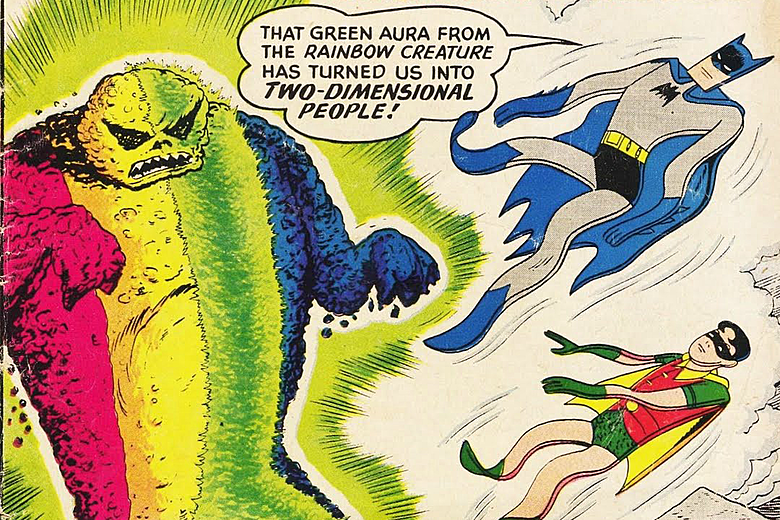The image is a detailed comic book page rendered in full color on an orange or beige background. Dominating the scene is a wide, fat monster with a round face divided into yellow and green halves. The creature's menacing features include two upside-down black triangles for eyes, a triangular nose, and an open mouth that reveals sharp white teeth. The monster's multicolored body consists of red, yellow, green, and blue stripes, and it exudes a green aura. This aura is pivotal to the scene as Batman, at the top right, explains in a speech bubble: "That green aura from the rainbow creature has turned us into two-dimensional people." Batman, clad in his signature black, gray, and blue costume, appears flattened and pushed backward. Below him is Robin, dressed in red, green, and yellow, also flattened, indicating their struggle against this enormous adversary. The image captures a moment of distress and urgency, as the heroes face the challenge posed by the formidable rainbow monster.